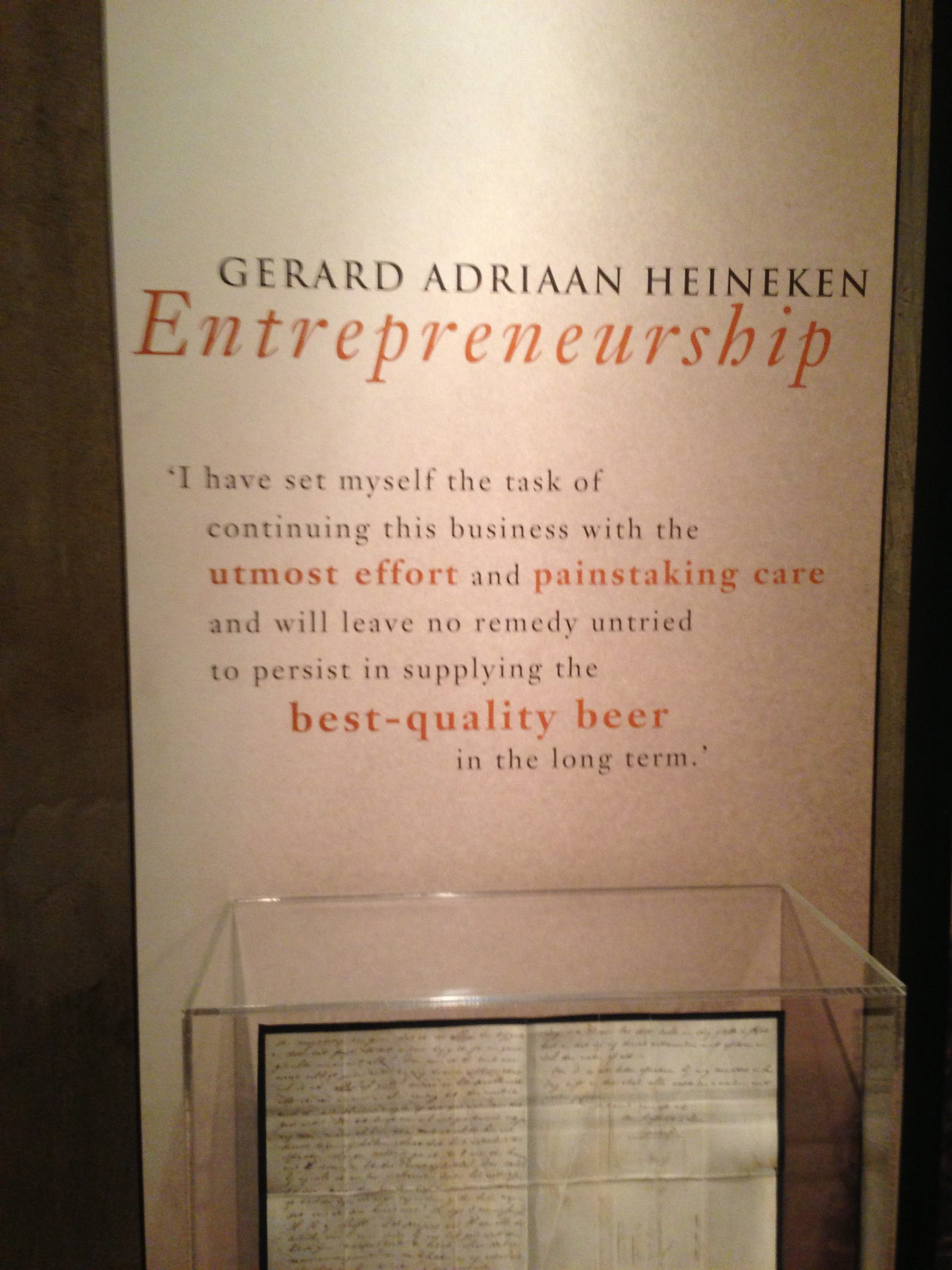The image is a detailed photograph, taken in portrait orientation, depicting an informational display at what seems to be a museum. The focal point of the display is a white banner with both black and orange text. The banner prominently features the name "Gerard Adrian Heineken" in black, followed by the word "entrepreneurship" in bold, italic orange text. Beneath this, a quote in black text reads, "I have set myself the task of continuing this business with the utmost effort and painstaking care and will leave no remedy untried to persist in supplying the best quality beer in the long term," with the phrases "utmost effort," "painstaking care," and "best quality beer" highlighted in orange. 

Below the banner, there's a protective plexiglass box containing an aged booklet, suggestive of a historical document, possibly related to the Heineken Beer Company. The booklet appears to be handwritten with several lines of text, spread over what looks like two pages and showing signs of having been folded. The display is illuminated by soft lighting, enhancing the visibility of both the banner and the contents within the glass box.